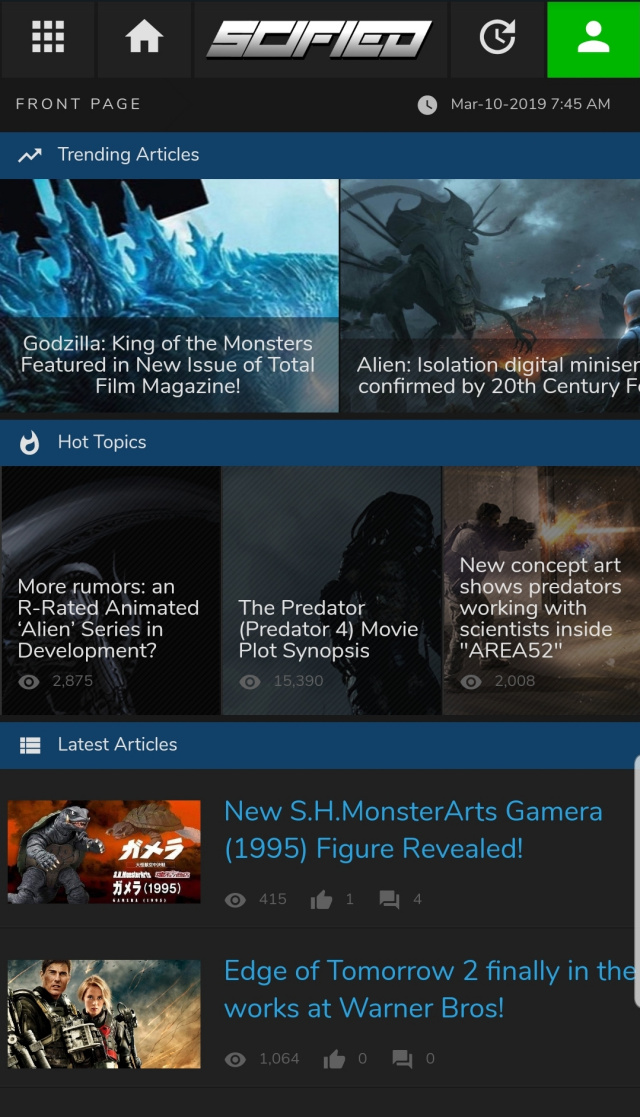**Detailed Caption:**

This image depicts a rectangular portrait screen capture, likely from a tablet or a cell phone, featuring a dynamic and visually rich website interface against a predominantly black background.

*Top Header:*
- The header at the top of the screen is very dark gray, slightly lighter than the rest of the background.
- To the far left is a grid icon consisting of nine small white rectangles arranged in a 3x3 formation.
- Next to the grid icon is a white house icon.
- Centered in the header is the website name "SciFied," written in a bold, blocky, stylized font that leans slightly to the right. The font is a silvery white.
- To the right of the website name is a refresh icon resembling the hands of a clock within a circular arrow.
- In the far right corner is a bright green square with a white user icon, representing a head and shoulders.

*Sub-header:*
- Beneath the header, the background turns black. On the left side in white all-caps font, it says "FRONT PAGE."
- To the right of "FRONT PAGE," there is a white clock face icon displaying black clock hands.
- Next to the clock icon, the date is displayed in white font: "MAR-10-2019 7:45 AM."

*Content Section:*
- The main content is divided into sections with alternating dark blue header bars.

**Trending Articles (First Section):**
- The header bar contains an upward jagged arrow icon and the title "TRENDING ARTICLES" in white font.
- Below this are two landscape-oriented images:
  - The left image shows a blue sci-fi scene with sky and sea, featuring craggy elements. The overlay text reads "Godzilla: King of the Monsters featured in new issue of Total Film Magazine!" in center-justified white font.
  - The right image depicts a sci-fi scene with an alien, dark clouds, and fire. The overlay text reads "Alien: Isolation Digital Miniseries Confirmed by 20th Century F...," with the final letters cut off.

**Hot Topics (Second Section):**
- The header bar features a flame icon and the title "HOT TOPICS" in white font.
- Below are three portrait-oriented images:
  - The left image has the text "More Rumors: An R-rated animated 'Alien' series in development?" with an eye icon indicating 2,875 views.
  - The middle image reads "The Predator (Predator 4) Movie Plot Synopsis" with a view count of approximately 25,000 or 35,000.
  - The right image displays "New concept art shows predators working with scientists inside 'Area 52'" with 2,008 views.

**Latest Articles (Third Section):**
- The header bar contains an icon resembling three rows of two squares and the title "LATEST ARTICLES" in white font.
- Below this are two full-color images:
  - The upper image showcases an orange background with a monstrous turtle, titled "New S.H. Monster Arts Gamera (1995) Figure Revealed!"
  - The lower image features a man and a woman in space armor with a mixed fiery yellow and blue sky background. The text reads "Edge of Tomorrow 2 finally in works at Warner Bros.!"
  - Each image is accompanied by three standard social media icons, including a gray thumbs-up for "like."

This detailed caption thoroughly outlines the visual and textual elements of the busy webpage, providing insight into its sci-fi themed content and structure.